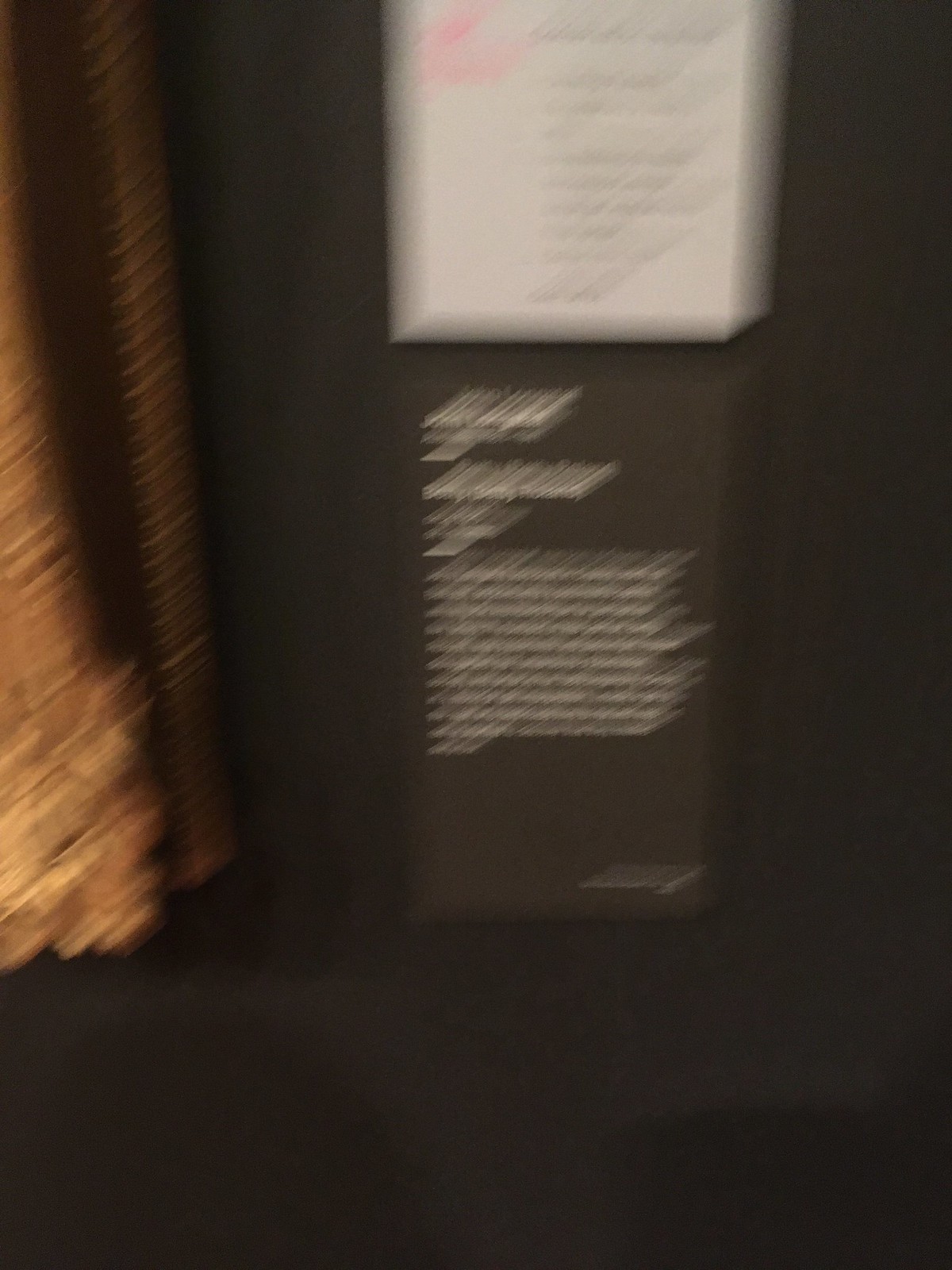The image depicts a dark brown wall adorned with a variety of elements. On the far left, there appears to be an object framed in gold and burgundy, though its details are indistinct due to the blurriness of the photo. Towards the middle at the top, there is a white paper with some pink markings which could be a drawing, label, or emblem on its left side, accompanied by extensive writing that continues down the page. Below this, a long piece of brown paper is visible, containing four paragraphs of white text. However, due to the lack of clarity in the image, the specifics of the writing remain unreadable.